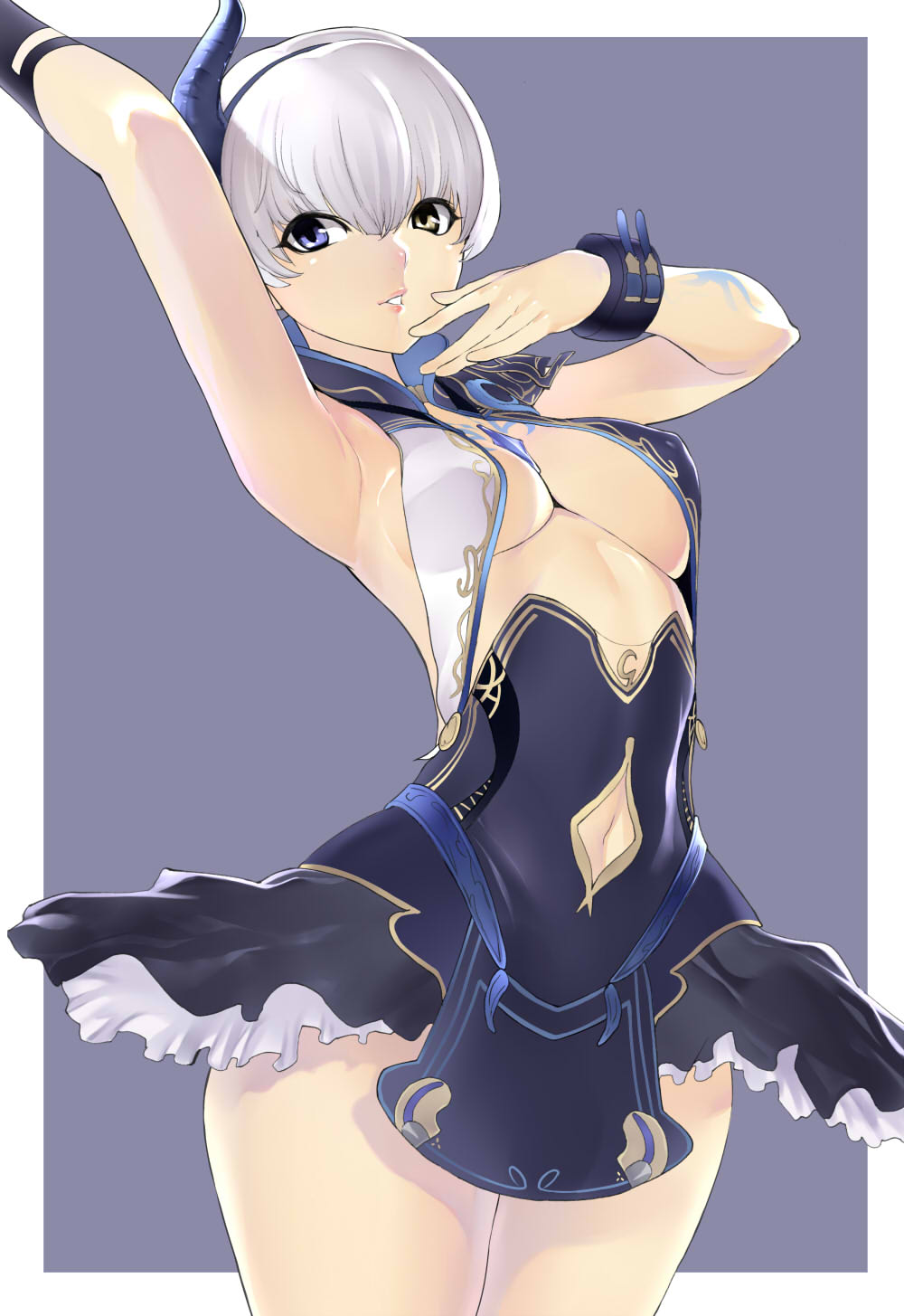The image is a detailed, digitally created anime-style drawing of a scantily clad woman standing against a plain, purplish background. The central character has short purplish-white hair adorned with a blue headband, and she is posed with one arm raised above her head, slightly leaning against it, while her other hand touches her chin. Her large eyes, small nose, and square chin are prominent features of her face. She is dressed in a revealing, dark blue-purplish dress with white frills and golden inlining around the hems. The dress is designed with two straps that cover her breasts and go over her shoulders, exposing her midriff, thighs, and legs. She wears black bracelets on her wrists. The entire composition appears artistic and could be part of a comic book, video game poster, or similar media. The image contains no text.